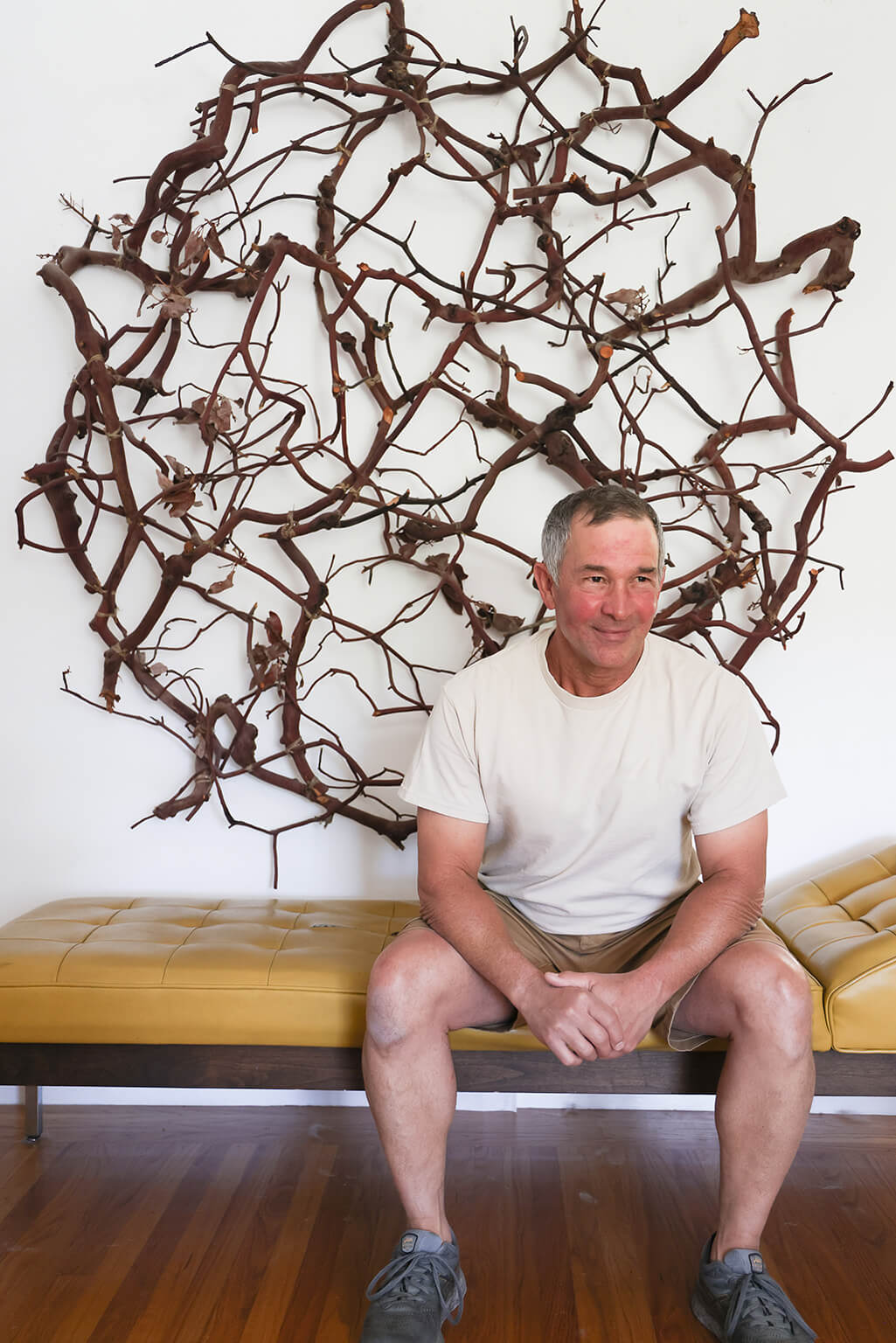This photograph captures an older white man with a light skin complexion seated on a long, light brown upholstered chaise lounge with a dark wooden base. The man, sporting salt and pepper hair and rosy cheeks with ears that protrude slightly, is smiling warmly and gazing off to the right. Dressed casually in a short-sleeved white t-shirt, short brown shorts, and black shoes with blue tongues, his feet rest comfortably on a wooden floor. Behind him, adorning the white wall, is an intricate piece of natural art—a large, circular arrangement of twisted, overlapping branches in various shades of brown, some still adorned with small brown leaves. The well-lit area provides a clear view of the scene, highlighting the craftsmanship of the branch sculpture and the serene demeanor of the man, who seems to take pride in or perhaps even credit for the creation behind him.